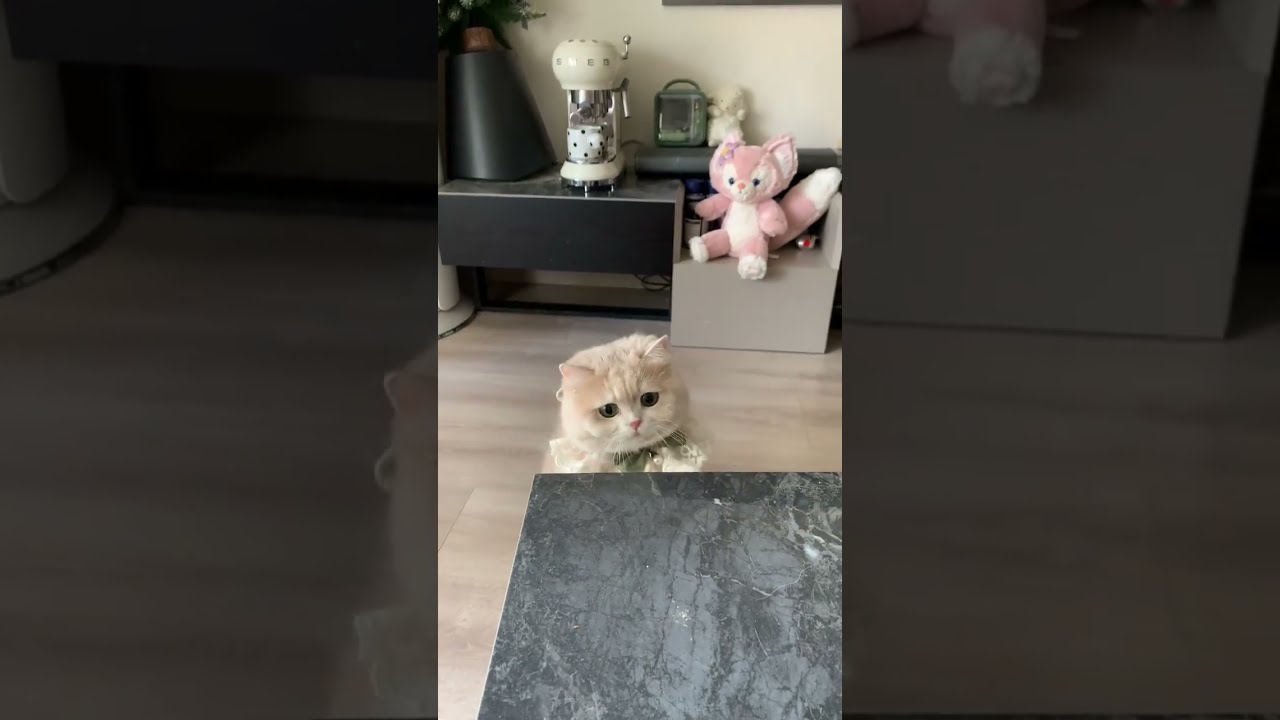The image is a wide, rectangular triptych with the left and right panels showing darker, magnified close-ups of the center image. The brighter central image features a fluffy beige and white cat with a pink nose and a green and white lace bow, captured from an above perspective. The cat sits next to a black and gray marble table, gazing up at it with wide, expectant eyes. Behind the cat is a beige wooden floor, a white espresso machine, and a shelf displaying a stuffed pink and white cartoon-like fox with a large tail. An unidentified black cone-shaped object with a brown cap appears in the top left corner of the image, reflecting some light. The cat's detailed features, the marble counter, and the surrounding household items contribute to a cozy, yet slightly melancholy atmosphere, possibly suggesting the cat is waiting for food.